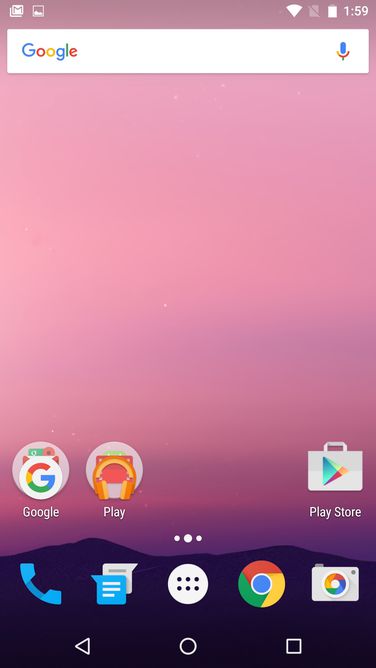The image showcases a screenshot of a smartphone's home screen. The background features a serene landscape with two small, dark purple hills or mountains situated at the bottom sixth of the image, creating a calm and minimalistic foreground. Above this, the remaining space is dominated by a captivating pink sky, accented with soft blue and purple hues, giving it a dreamy and ethereal appearance.

In the middle section of the screen, various application icons are neatly arranged. Notable apps include Gmail and Google Photos, which are easily identifiable among others. Above the app icons, a Google search bar is prominently displayed.

At the very top of the screen, the time is displayed as 1:59, alongside standard status icons such as the battery indicator and connectivity symbols. 

The bottom of the interface houses a navigation bar with essential buttons for Google, Google Play, Play Store, the phone dialer, the main menu, possibly another Google app, Google Photos, and a documents app.

The overall appearance is organized and functional, with a visually appealing background that adds a touch of elegance to the user's interface.